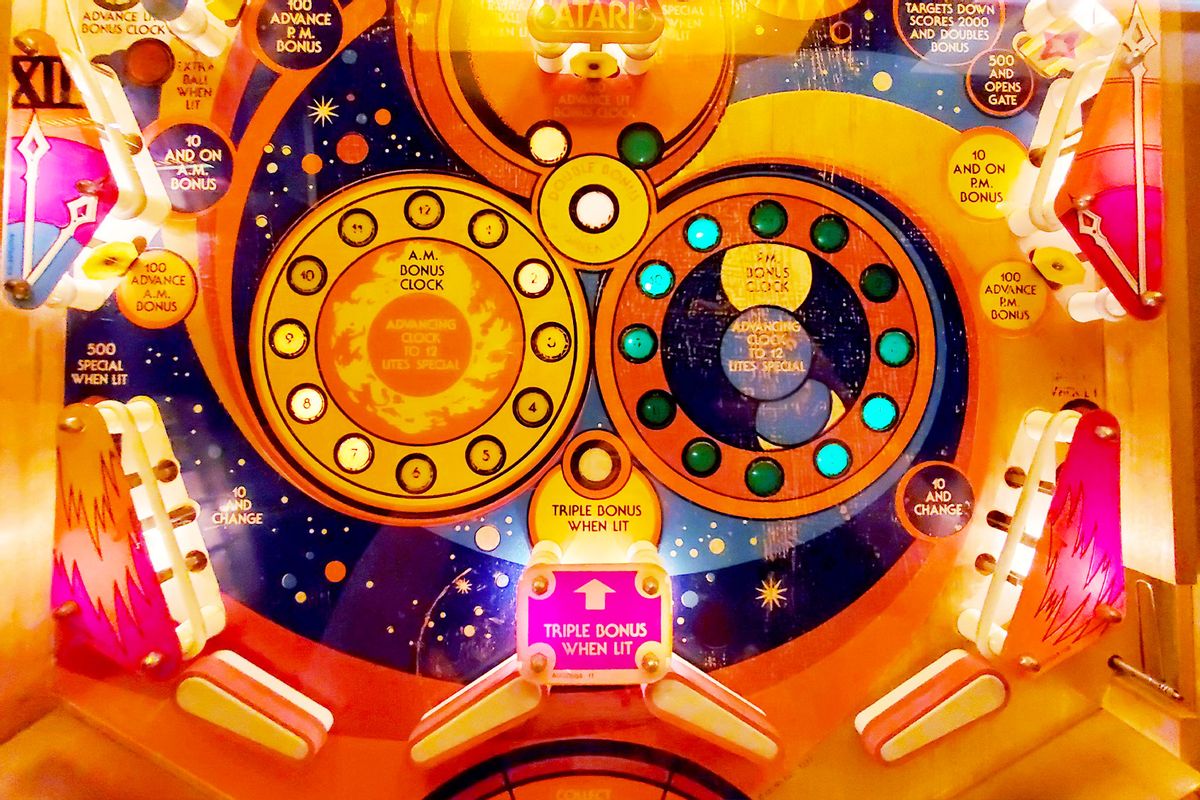The image depicts a vibrant and colorful pinball machine viewed from an overhead perspective. The design prominently features an engaging space motif, with a dark blue background adorned with planets, stars, and cosmic elements in vivid oranges, yellows, and blues. Toward the bottom of the machine, you see orange and yellow flippers, which are the paddles used to hit the ball. Various sections of the machine are inscribed with phrases like "100 Advance AM Bonus," "500 Special When Lit," "Targets Down Scores 2000 and Doubles Bonus," and "10 and On PM Bonus." The machine also displays the term "Atari" at the top, confirming its retro theme. Small circles, potentially indicating different bonuses and specials, are scattered throughout the field. The entire setup, with its intricate illustrations and bright hues, evokes a classic arcade experience.